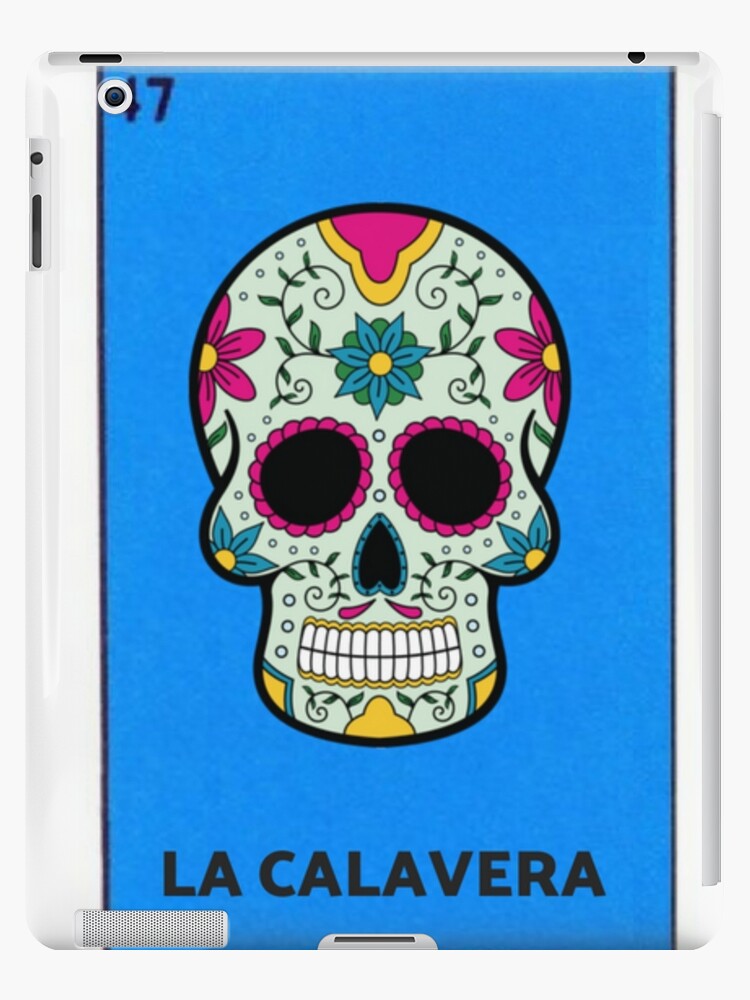This lively and intricate illustration portrays a vividly colorful sugar skull, reminiscent of the Grateful Dead style but not directly linked to it. The sugar skull, named La Calavera and adorned with floral decorations, symbolizes the Day of the Dead. Its vibrant detailing includes a base of pink flowers, gold borders, and various hues like blue, yellow, black, and pink. Against a bright blue background, the skull’s large, almost smiling teeth and hollow, black-outlined eyes present a playful rather than frightening visage. 

The top of the skull's head features a gold-trimmed pink skull, while the center of the forehead is adorned with vines and a blue flower with a yellow center. The eye sockets are accentuated with pink outlines, and at each cheekbone end, there's a blue flower with three petals and a yellow center. Below the hollow nose, two pink lines radiate outward. Below the teeth on the chin, a yellow upside-down lemon-shaped design is visible. "La Calavera" is inscribed in dark lettering at the bottom, tying the character to its cultural roots. Set within a clear case resembling a bingo card eye pad case, the design includes a numerical detail at the top left corner, where only the digit seven is visible due to a hole covering the other number.